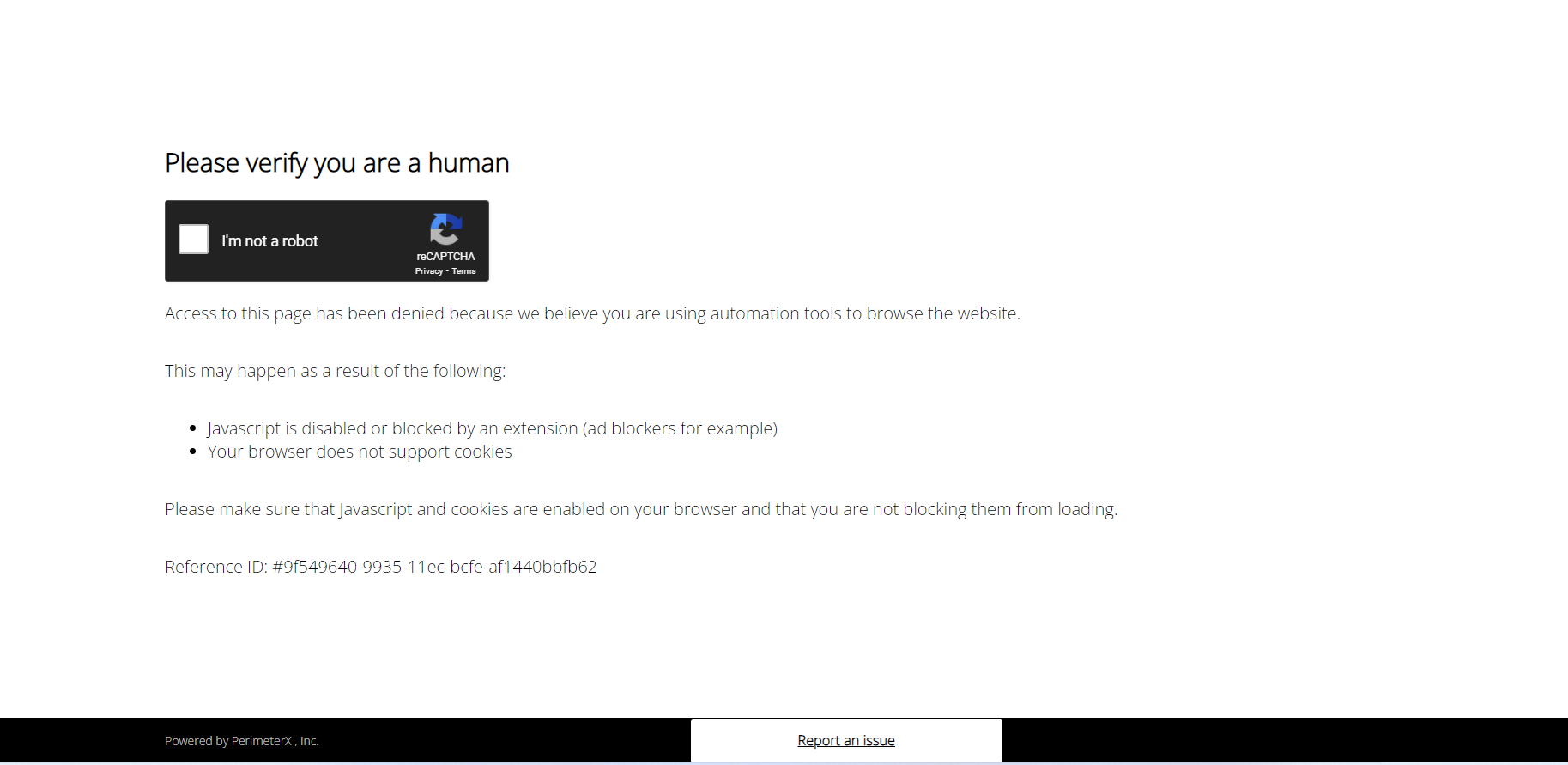This screen capture showcases a section of a website featuring a reCAPTCHA verification popup. The webpage has a clean, white background with black text predominantly aligned to the left side of the screen. Across the bottom of the image, there is a black banner containing small, white text on the left side that appears to read "Powered by possibly Perimeter Ink," though the low image resolution makes it difficult to decipher with complete certainty. 

Prominently displayed in the center of this black banner is a white button with the black text "Report an issue." On the upper part of the webpage, the largest and most legible text reads "Please verify you are a human," compelling the user to confirm their authenticity. Directly below this prompt, there is a black rectangular button bearing the reCAPTCHA logo, which consists of three circular arrows in shades of light gray, light blue, and dark blue. 

On the left side of the reCAPTCHA button, there is an unchecked white checkbox beside the phrase "I'm not a robot" in white text. Underneath this main section, there are a few lines of text, including two bullet points and a reference ID, which further contribute to the site's security verification process.